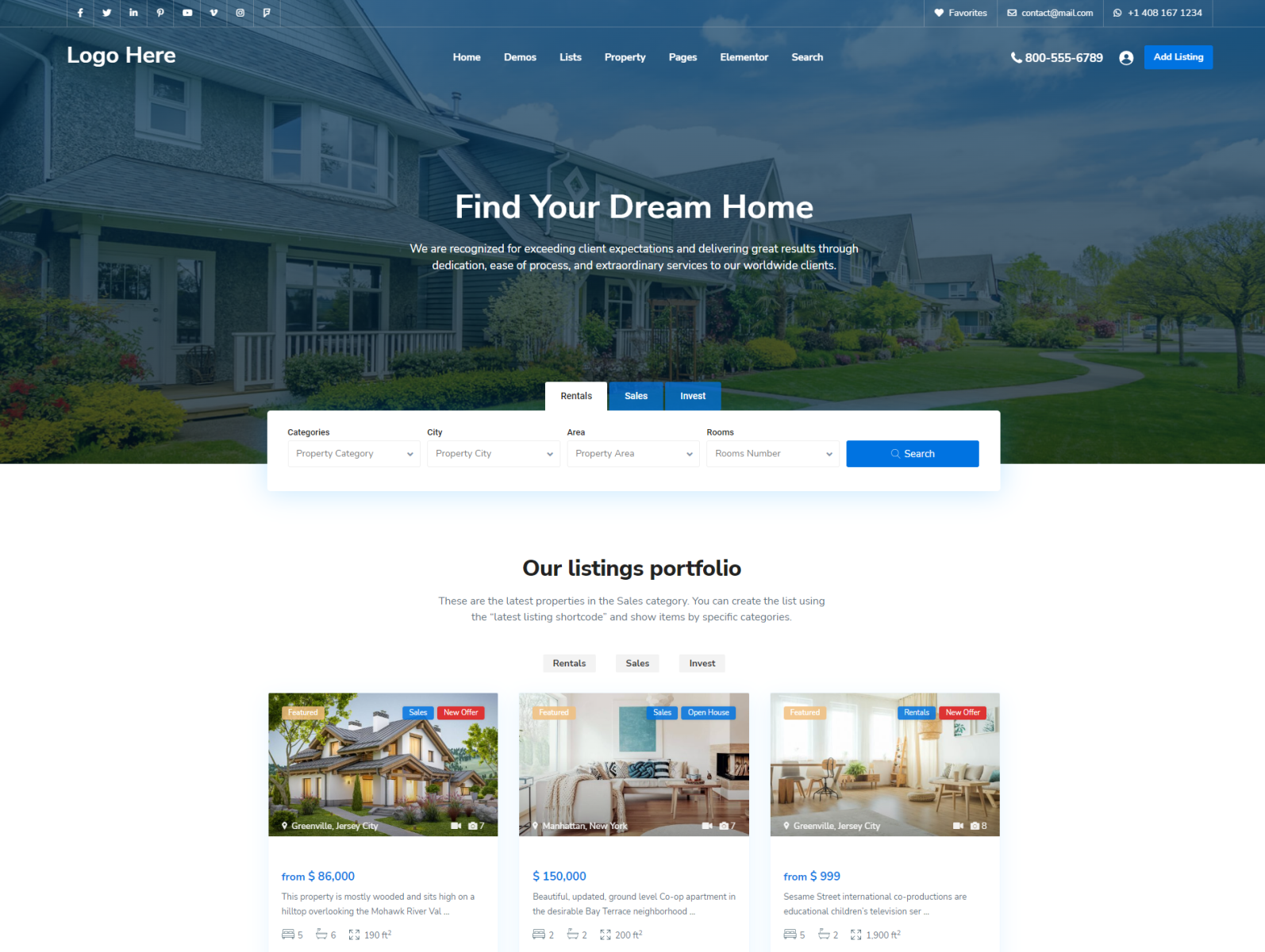This screenshot features a meticulously designed landing page for a real estate website. The focal point of the banner is a picturesque image of a serene neighborhood, showcasing lush trees and neatly aligned houses, each with a well-maintained front yard. On the left-hand side of the banner, various social media icons are displayed prominently.

Centered at the top, the page is marked with a placeholder for the company logo, flanked by a horizontally arranged navigation menu. This menu includes links to essential sections: Home, Property Listings, and Additional Resources. On the upper right-hand corner, there is contact information, prominently featuring a phone number, as well as options to log in or get in touch with the company.

Below the banner, set against a white background, is a navigation bar designed for easy browsing. When expanded, this navigation bar appears in white, offering various search categories for users to input their preferences. Accompanying the search feature are two distinct blue buttons for additional actions.

Further down the page, a section titled "Our Listings" showcases a portfolio of properties, each presented with a high-resolution image. Each listing includes crucial details such as the price, the number of bedrooms, and other relevant data, allowing potential buyers to quickly gauge if a property meets their criteria.